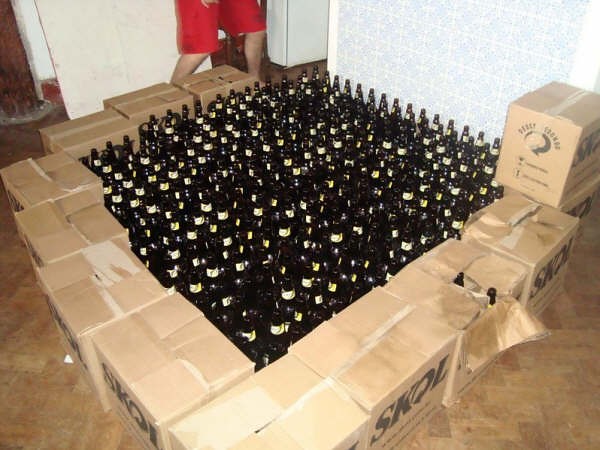The photograph captures an indoor setting, possibly a room in a rented house or dorm, featuring an elaborate display of over 100 empty beer bottles. These dark brown or black bottles with tan labels on the neck are meticulously arranged in neat rows and columns, forming a square inside a perimeter of brown boxes. The boxes, marked with the letters "SKOL," are of the same height as the bottles and create a border around the display, suggesting a resemblance to a carnival ring toss game setup. The herringbone pattern of the synthetic wood floor and the off-white walls frame this scene. In the background, a young person wearing red sports shorts stands, with their bare legs visible, adding a human element to the composition.